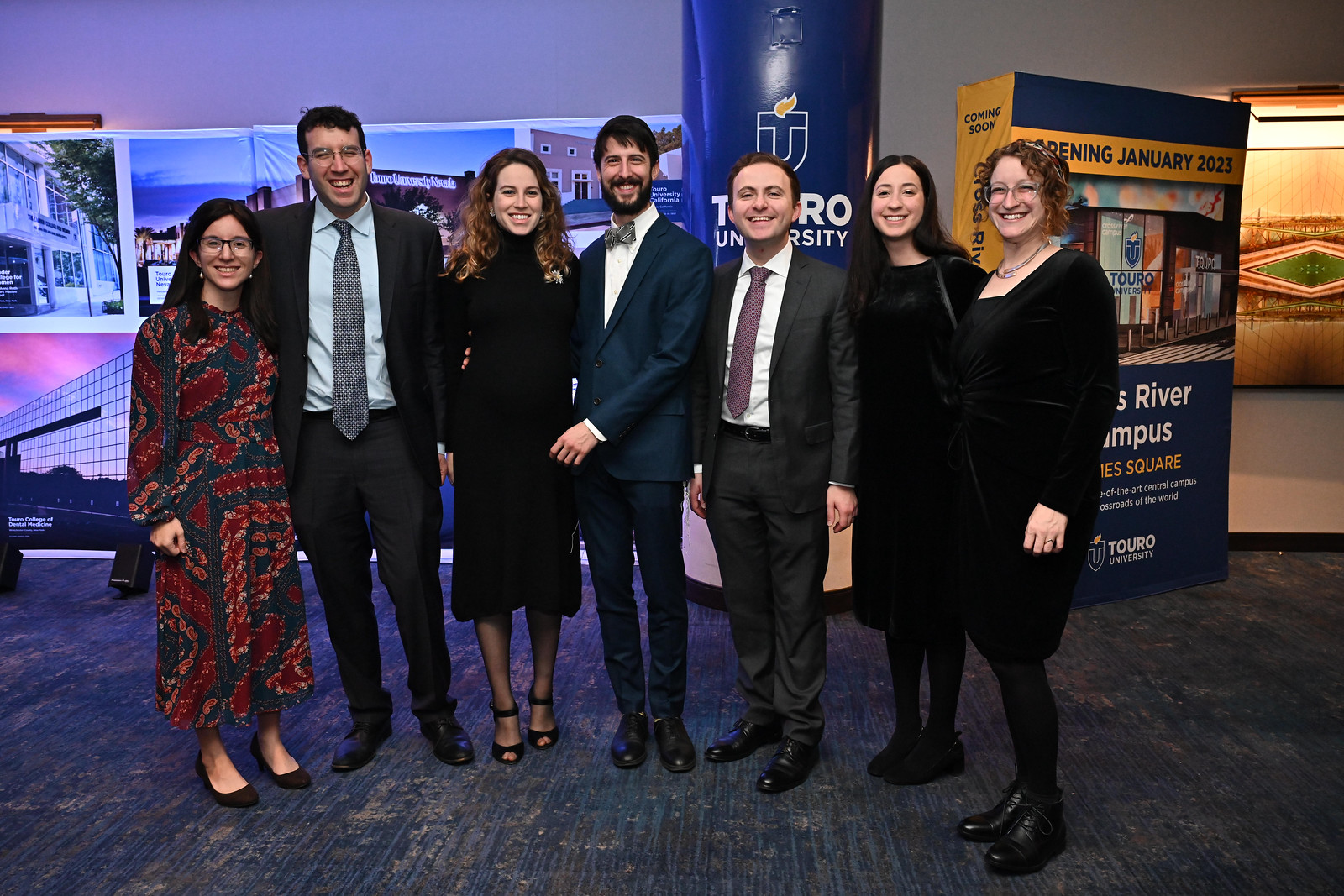A group of seven professionally dressed individuals, consisting of three men and four women, are standing in a carpeted room adorned with signage and backdrop elements from Touro University, indicating an official event or reception. The men are attired in dark suits, button-down shirts, and ties, while the women sport elegant dresses, predominantly black, with one woman in a distinctive red and black dress. The light purple walls on the left and the blue lighting cast a sophisticated ambiance, highlighting various images and signs behind them, one of which proclaims "Opening January 2023" with mention of "campus." The setting resembles a convention center or similar professional gathering space.